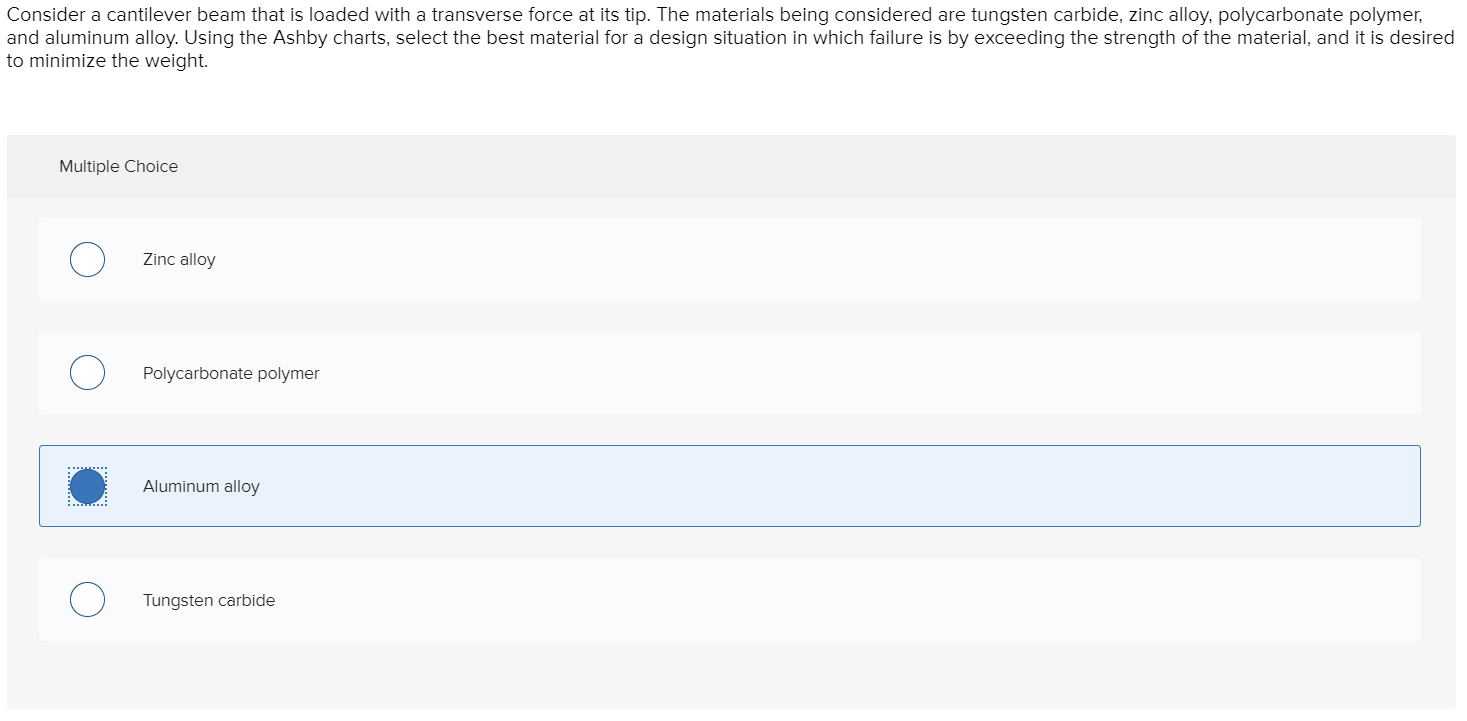The image is a detailed screenshot of a multiple-choice question related to material selection for a cantilever beam subject to a transverse force at its tip. The background is predominantly white with black, computer-typed text. At the very top of the screen, the question reads: "Consider a cantilever beam that is loaded with a transverse force at its tip. The materials being considered are tungsten carbide, zinc alloy, polycarbonate polymer, and aluminum alloy. Using the ASPE charts, select the best material for a design situation in which failure is by exceeding the strength of the material, and it is desired to minimize the weight."

Directly below this question, a multiple-choice box is displayed against a slightly lighter gray background. The label "Multiple Choice" is positioned at the top of this box. Within the box, there are four selectable options, each accompanied by a clickable circle for selection. The options are listed as follows:
1. Zinc alloy
2. Polycarbonate polymer
3. Aluminum alloy (outlined in blue to indicate that this is the selected answer)
4. Tungsten carbide

The detailing of the choices and the highlighted selection underscore the user's decision-making process when determining the most suitable material for the given engineering scenario.